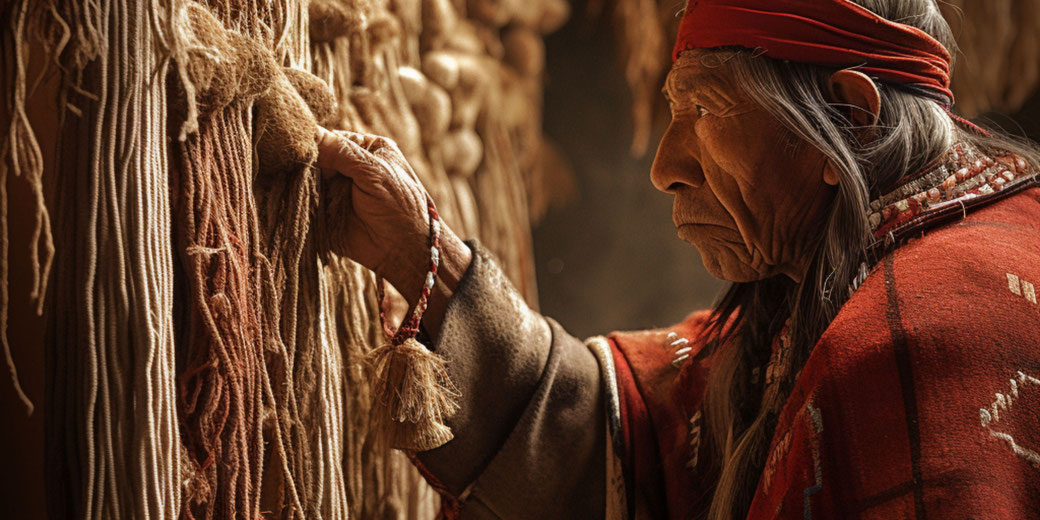The horizontally aligned rectangular image showcases an elderly Native American man, characterized by his deeply wrinkled skin, large nose, and long gray hair. He wears a red headband that complements his traditional heavy-looking red robes adorned with tan and white Native American patterns. The man has a serious yet focused expression, with the corners of his mouth turned slightly downward, possibly indicating concentration rather than sadness. His right hand is raised, interacting with thin, brown strings or ropes hanging from a dark, blurry background that resembles a stone wall. He appears to be selecting one of these threads, suggesting he might be engaged in a craft or traditional activity, possibly related to textile making. The scene is detailed with his attire extending to a wristband twisted in red and white colors, adding to the cultural richness of the image.